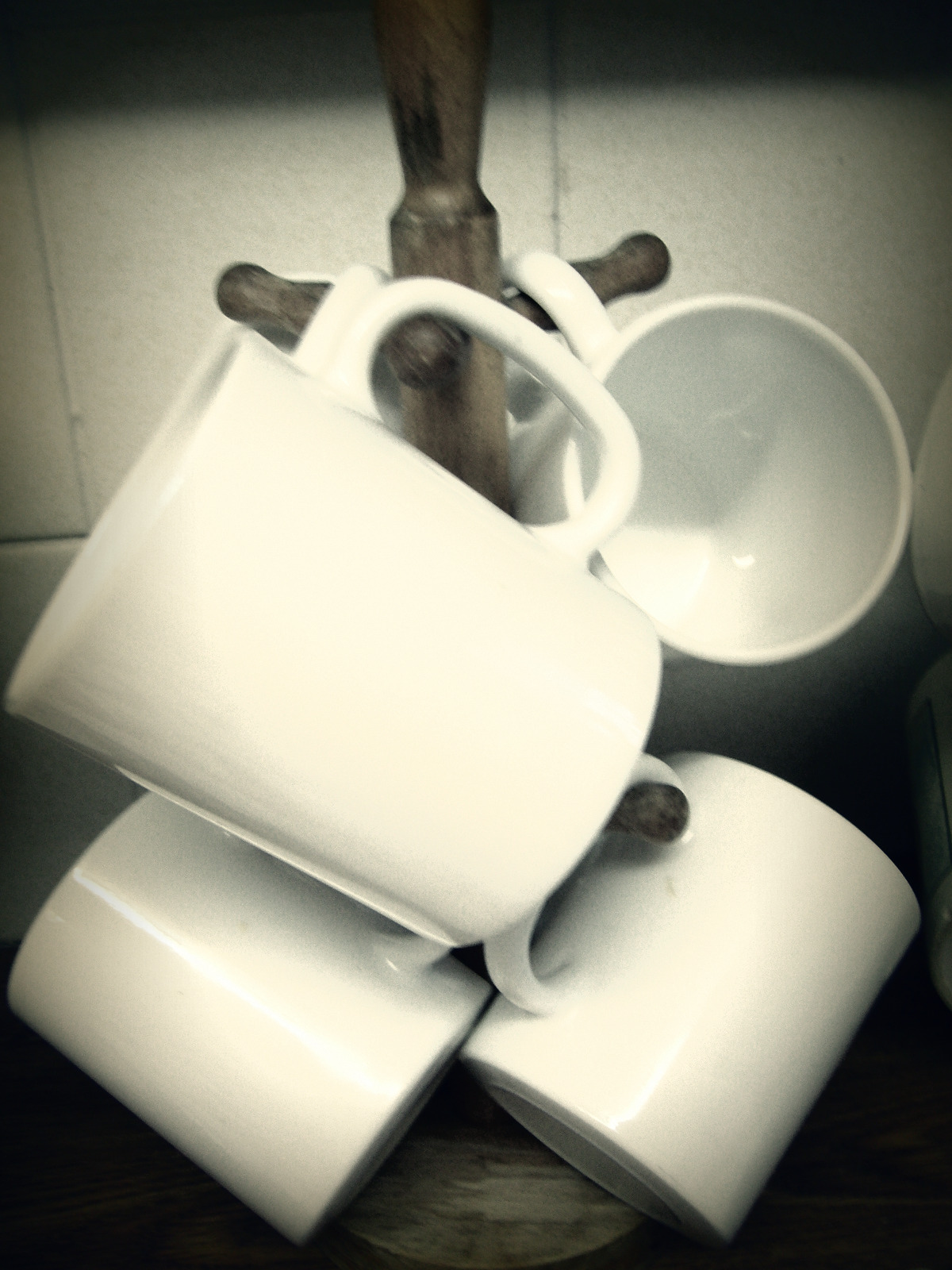This detailed photograph captures a wooden coffee mug holder placed in a kitchen setting. The holder is made from dark brown wood and features a single vertical stake with several small pegs designed to hold coffee cups. There are six pristine, white coffee mugs hanging from the pegs, each devoid of any text or images. The kitchen background is adorned with a rectangular, off-white tile backsplash, separated by white grout. A wooden countertop, matching the color of the mug holder, runs beneath the holder, while a cabinet above casts a shadow that slightly darkens the scene. The clean, uniformly white mugs, with visible details from various angles, contrast gently with the rustic wood and neutral tiles, creating a cozy yet elegant kitchen vignette.